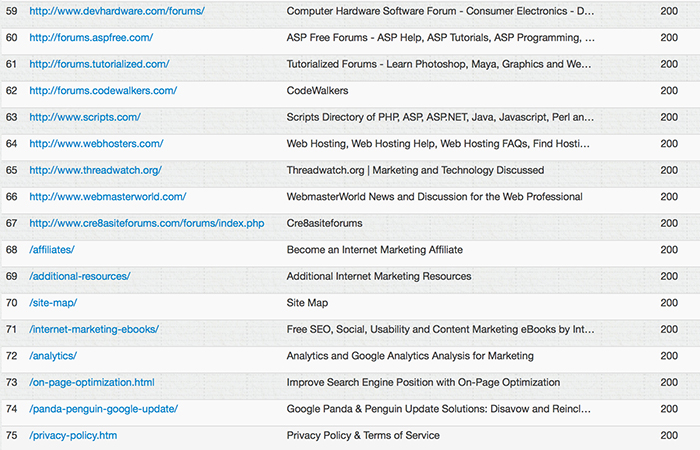This screenshot displays a table listing various subdomains or URLs, organized into three columns. The first column contains numerical identifiers, followed by the respective URLs. The second column consists of titles or descriptions corresponding to each URL. The third column consistently shows the number '200' alongside each entry. The numerical range for the listed items extends from 59 to 75. Notably, each entry is set against an alternating gray and lighter gray background, enhancing visual distinction. The URLs featured in this table include 'http://divhardware.com', 'http://forums.ascpfree.com', 'http://forums.tutorialize.com', 'http://forums.codewalkers.com', 'http://scripts.com', 'http://webposters.com', 'http://threadwatch.com', and 'http://webmasterworld.com'.